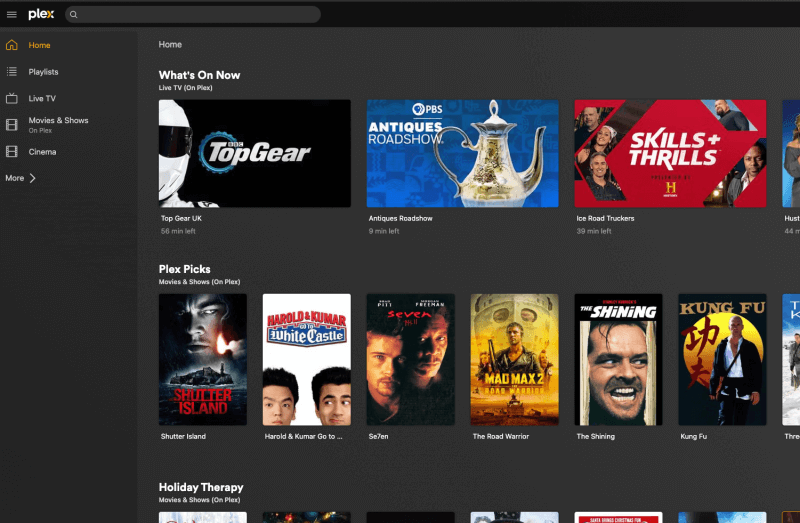The interface of the Plex streaming service is displayed. In the top left corner, the Plex logo is prominently featured, with the last letter partially in orange. Below the logo, the main navigation is visible, offering options such as Home, Playlists, Live TV, Movies & Shows, and Cinema.

Under the Home section title, the text "What's on now?" is displayed in white, showcasing current streaming options. Featured shows include "Top Gear UK," an image of a gold teapot for "Antiques Roadshow on PBS," and "Skills and Thrills: Ice Road Truckers."

The second row, titled "Plex Picks: Movies and Shows on Plex," highlights various movies. These include "Shutter Island," with a dark building on a secluded island and Leonardo DiCaprio holding a flame; "Harold and Kumar Go to White Castle"; "Seven," featuring Brad Pitt and Morgan Freeman; "Mad Max 2: The Road Warrior"; "The Shining," with Jack Nicholson peering through a door; and "Kung Fu," featuring a man silhouetted against a yellow sun.

At the bottom of the screen, only the title "Holiday Therapy" is partially visible, suggesting another category of curated content.